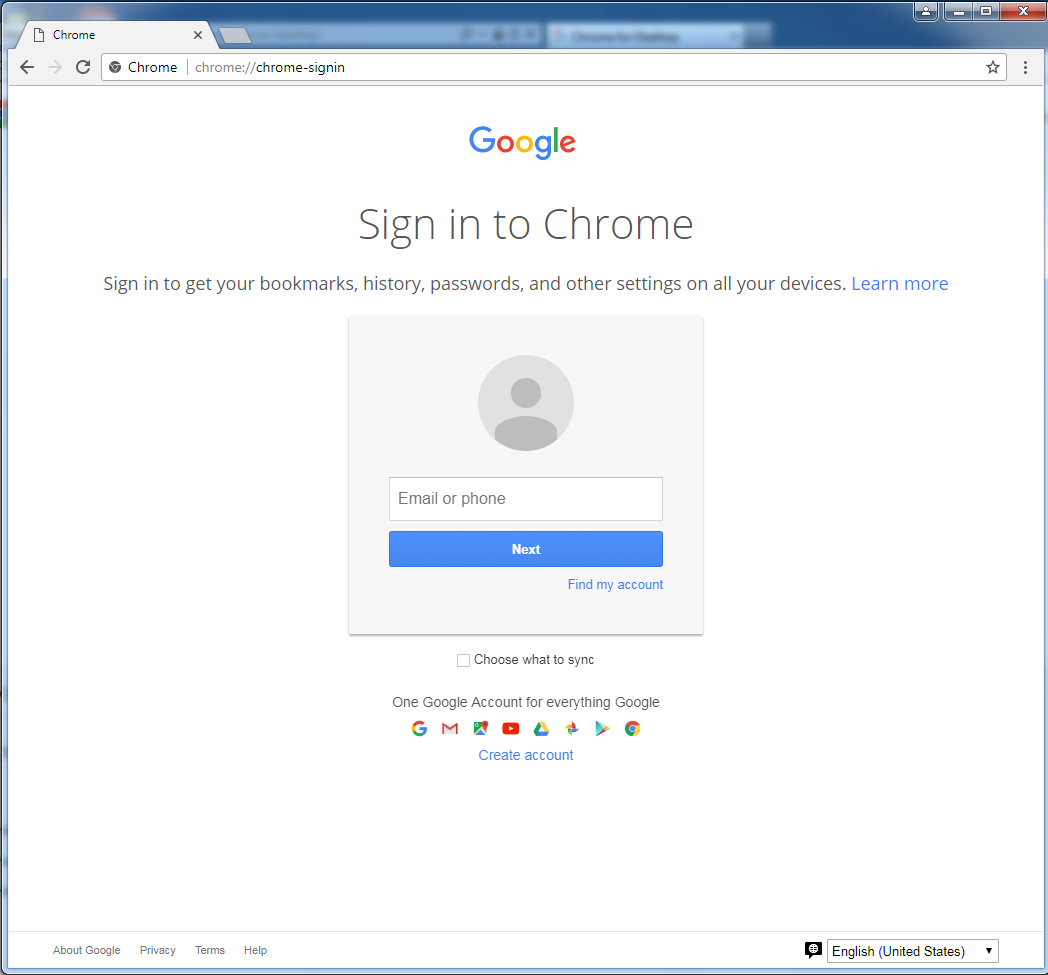This image captures a screenshot of the Google Chrome sign-in page. In the top-left corner of the browser, there is a single open tab, labeled "Chrome." Directly beneath the tab, there are navigation icons for backward, forward, and page refresh functions. To the right of these icons is the URL bar, displaying "chrome://chrome-signin."

At the top-right corner of the browser window, typical window control icons are visible: a red-background X for closing the window, a square for maximizing or resizing, and a dash for minimizing the browser window.

At the center-top of the image, the Google logo is prominently displayed, featuring the familiar multi-colored letters: blue “G,” red “O,” yellow “O,” blue “G,” green “L,” and red “E.” Below the logo is the headline, "Sign in to Chrome," followed by the description, "Sign in to get your bookmarks, history, passwords, and other settings all on your devices." A "Learn more" link is included in light blue text for additional information.

Beneath this text, there is a sign-in form. It features a square box with an icon shaped like a circle, denoting the input area for user credentials. Below this, there is a prompt for "Email or phone," indicating the field where users should enter their login information. Beneath this input field, there is a rectangular button with a blue background and white text that reads "Next," guiding users to proceed with the sign-in process.